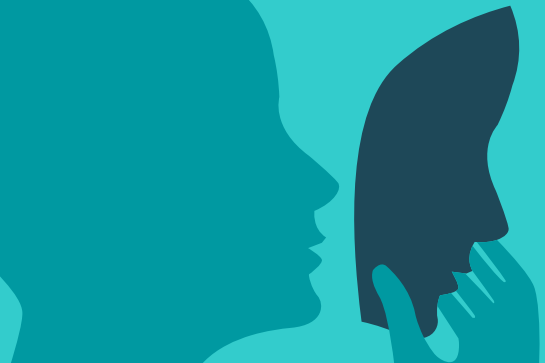The image is a simple yet striking graphic design in three colors, featuring a side profile of a person, likely of European descent, with distinctive thin nose and lips. This figure, which appears to be a woman given the delicate outline, is depicted in a dark teal color and is facing to the right. The person is holding a dark blue mask in front of their face with their right hand, as if about to put it on. The mask is shaped exactly like their face, emphasizing a duality or hidden identity theme. The background of the image is a lighter turquoise color, creating a subtle contrast that highlights the serenity and simplicity of the composition. The overall design lacks intricate facial features, eyes, or any other defining expressions, relying solely on block colors and clean contours to convey its message. There are no animals, mechanical objects, structures, or text, reinforcing the minimalist and abstract nature of the artwork.